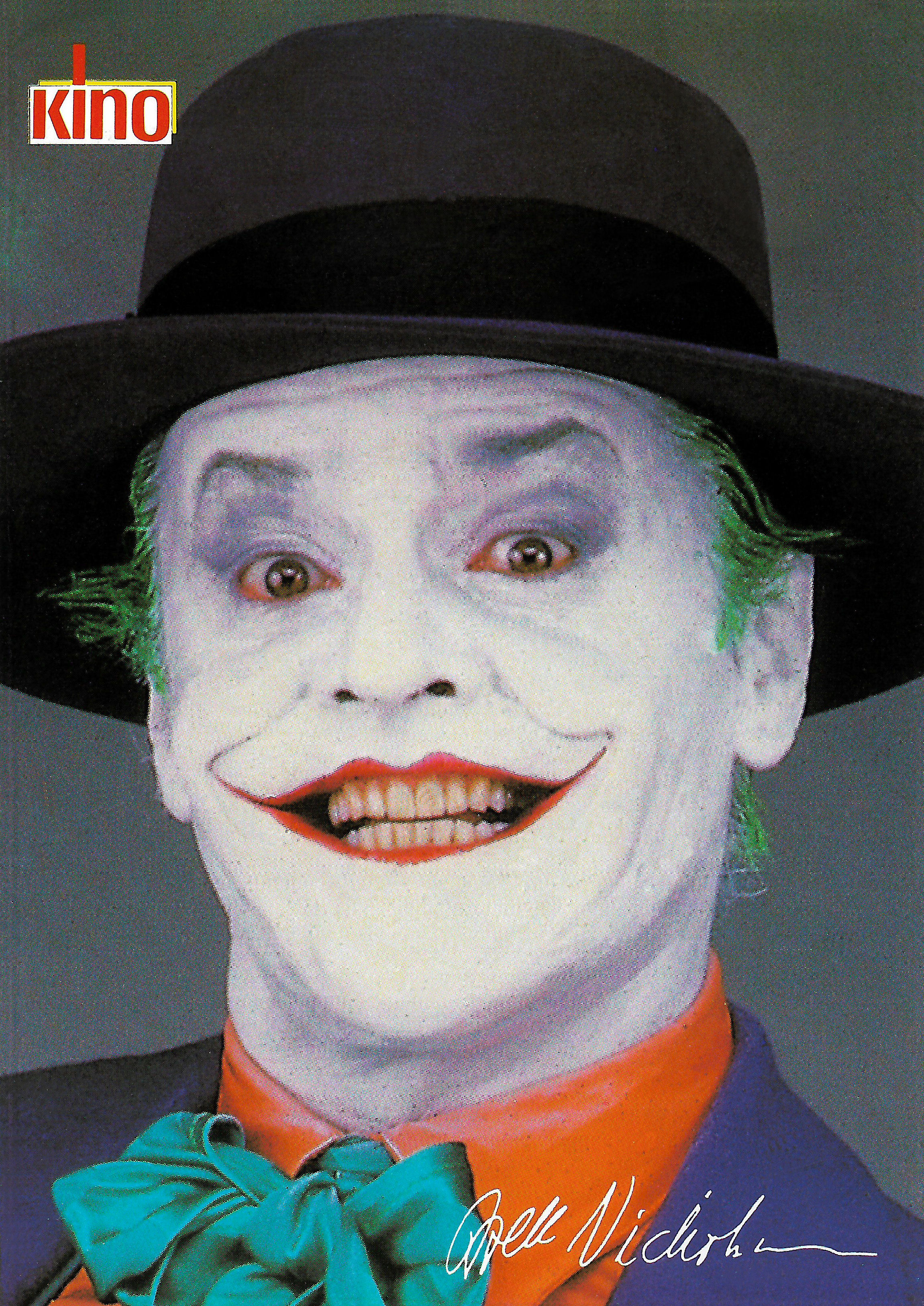This color photograph features Jack Nicholson famously dressed as the Joker, the iconic character from the Batman series. In the top left corner, there's a white logo with red lettering that spells "Kino," which might indicate a brand name, magazine title, or an advertisement. Nicholson's character is vividly brought to life with striking makeup: his face is painted a chalky white, with exaggerated, thin red lips and eye outlines, and distinctive green eyebrows and hair. He is adorned in a classic Joker ensemble, wearing a black hat with a felt ribbon, a red shirt, and a purple jacket. Completing his flamboyant look is a green ruffled bow tie. The photograph is a close-up, focusing solely on his face and upper torso, with his signature, "Jack Nicholson," penned in white at the bottom of the image.